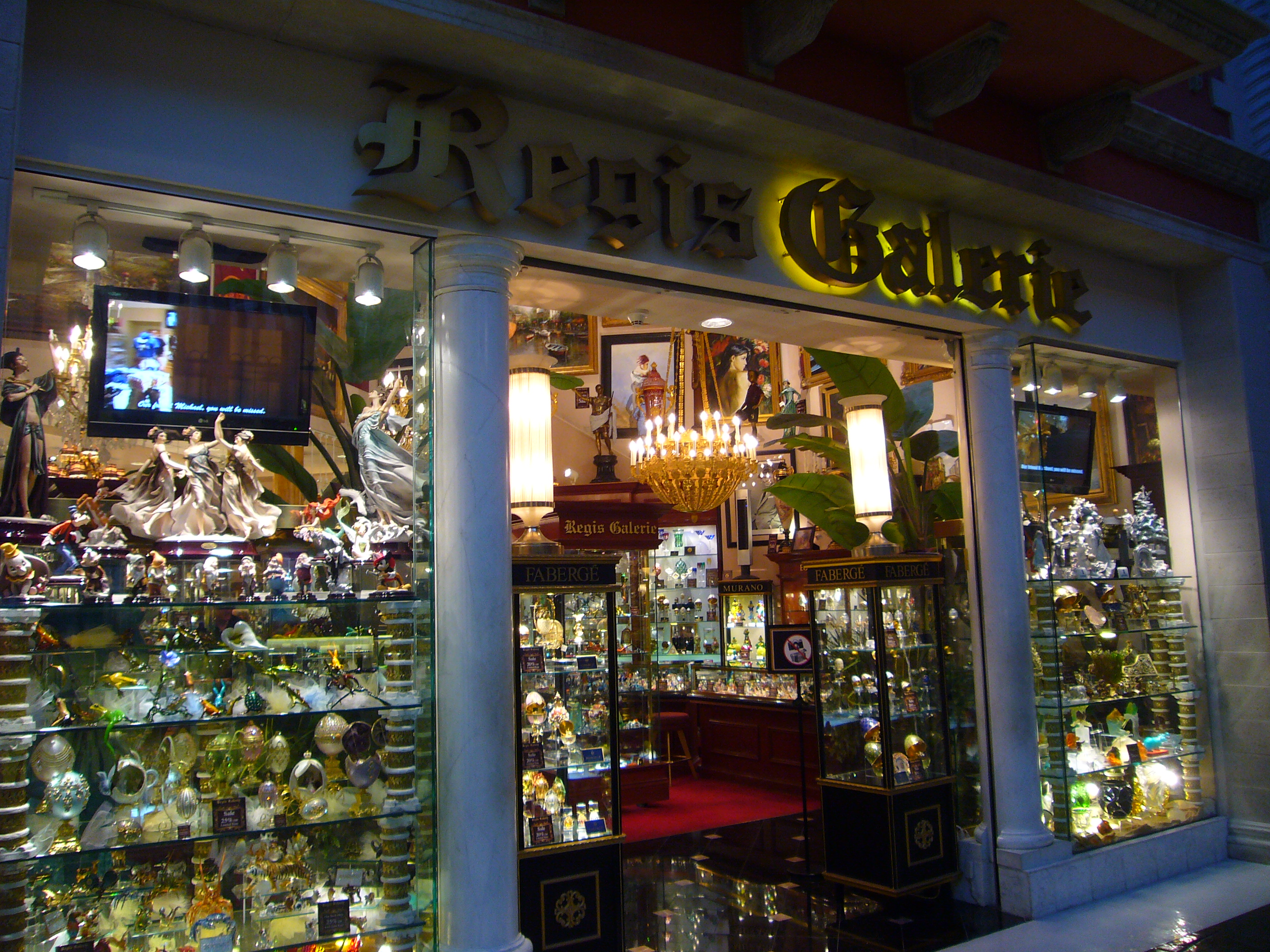The image depicts a pristine white storefront of a shop named 'Regis Galerie,' as indicated by the gold-lettered sign at the top. The word 'Galerie' is illuminated with a warm yellow backlight, while 'Regis' remains unlit. The entrance is flanked by two elegant white pillars and flanked by large glass display windows showcasing an array of crystal eggs, ornate figurines, and various trinkets positioned on glass shelves. The interior, visible through the center doorway, reveals a luxurious setting with a gold chandelier hanging centrally, accompanied by two gold pillar lights on either side. The store's floor transitions from glossy black in the foreground to red carpeting further inside. The interior is lined with glass display cases cluttered with similar eclectic and decorative items, and there's a TV in the upper left corner of the shop. The overall aesthetic is one of opulence and intricate detail.